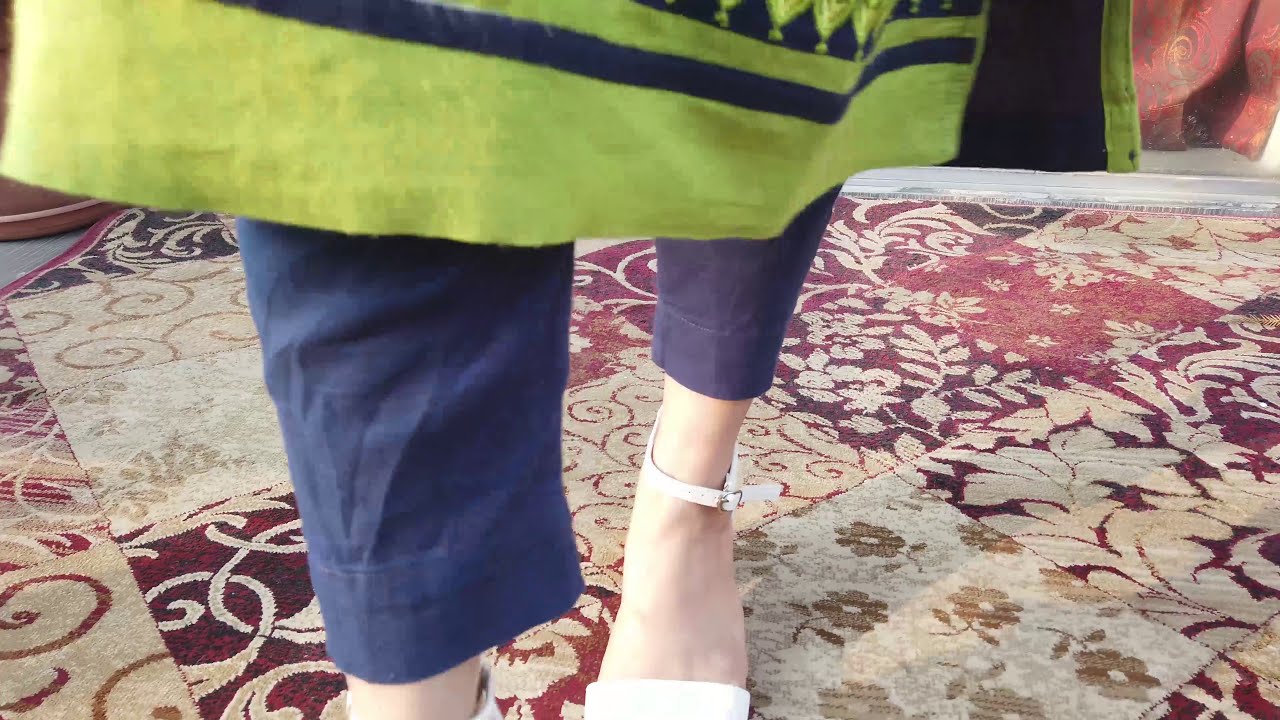A white woman stands on an intricately designed, somewhat worn tan and burgundy rug, which features a variety of detailed square tiles adorned with floral and scrollwork patterns. The colorful patchwork rug appears to be in a marketplace setting. The woman's outfit includes moderately fitting blue pants reaching the top of her ankles and white sandals with ankle buckles. Visible portions of her attire also reveal a long shirt or dress with green and black elements, including two horizontal black lines. Only her right foot and part of her dress are prominently displayed from the given perspective.